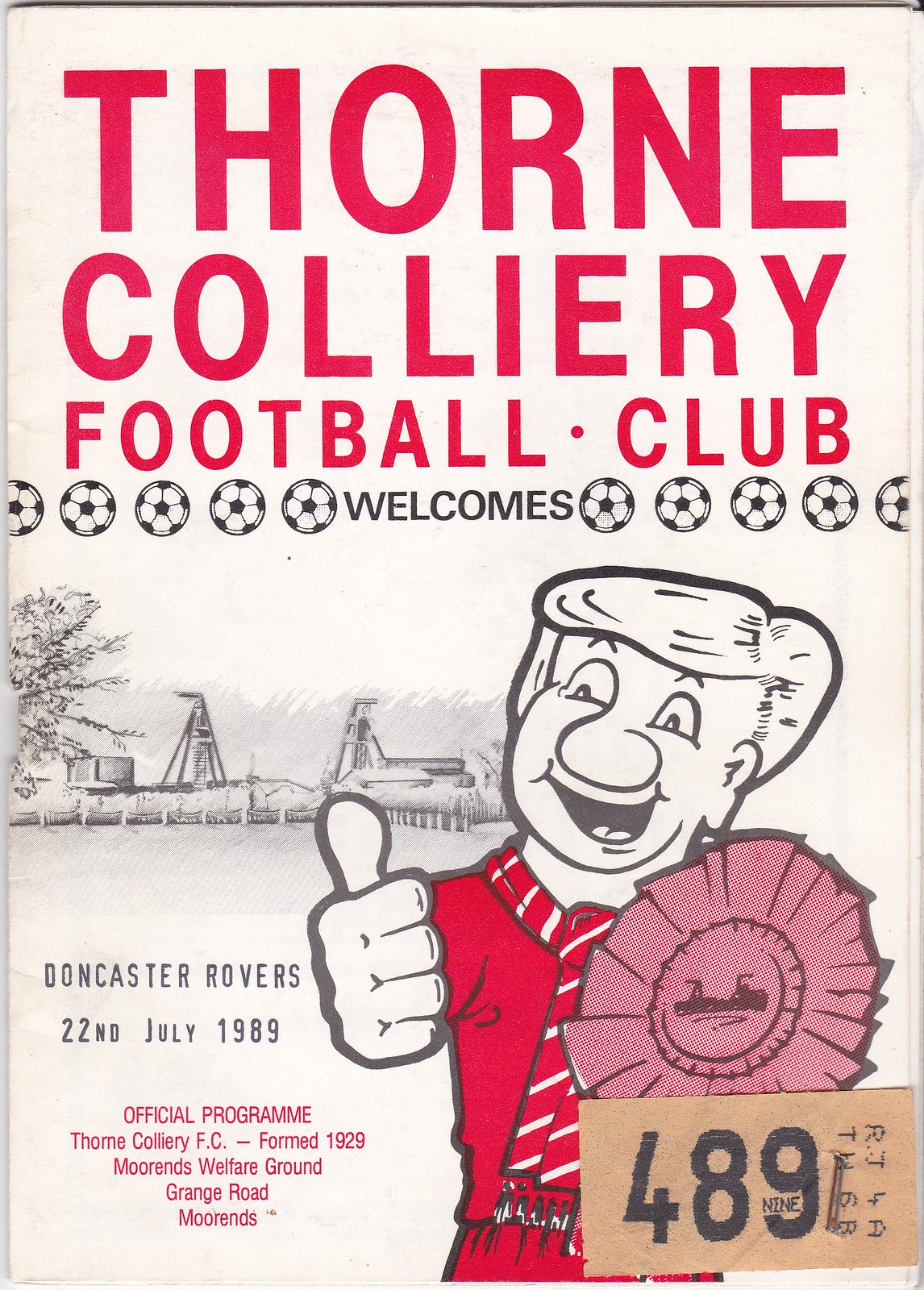The image is a photograph of an official program from a soccer match between Thorn Colliery Football Club and Doncaster Rovers, dated 22nd July 1989. The cover of the program is off-white and rectangular, indicating its age with a slightly worn appearance. At the top, in bold red text, it announces "Thorn Colliery Football Club Welcomes Doncaster Rovers." The word "welcomes" is flanked by small soccer ball icons. Below this, significant text confirms the details: "Official Program, Thorn Colliery FC, formed 1929." The venue information is partially legible but mentions Moran's Welfare Ground on Grand Road.

Prominently featured on the bottom right area of the cover is a cartoon character with a thumbs-up gesture, dressed in red attire that includes a shirt, shorts, and a possibly striped neck scarf or muffler. This character, which some suggest resembles a cartoon version of Donald Trump, stands against a backdrop that includes buildings and a large pink rosette. To the right of this character is a blue and brown box marked with the number 4899, possibly a staple or additional numbering. Additional details include a ribbon and mentions of a possible copyright re-illustration error. The overall design reflects a historic and communal sports event program.